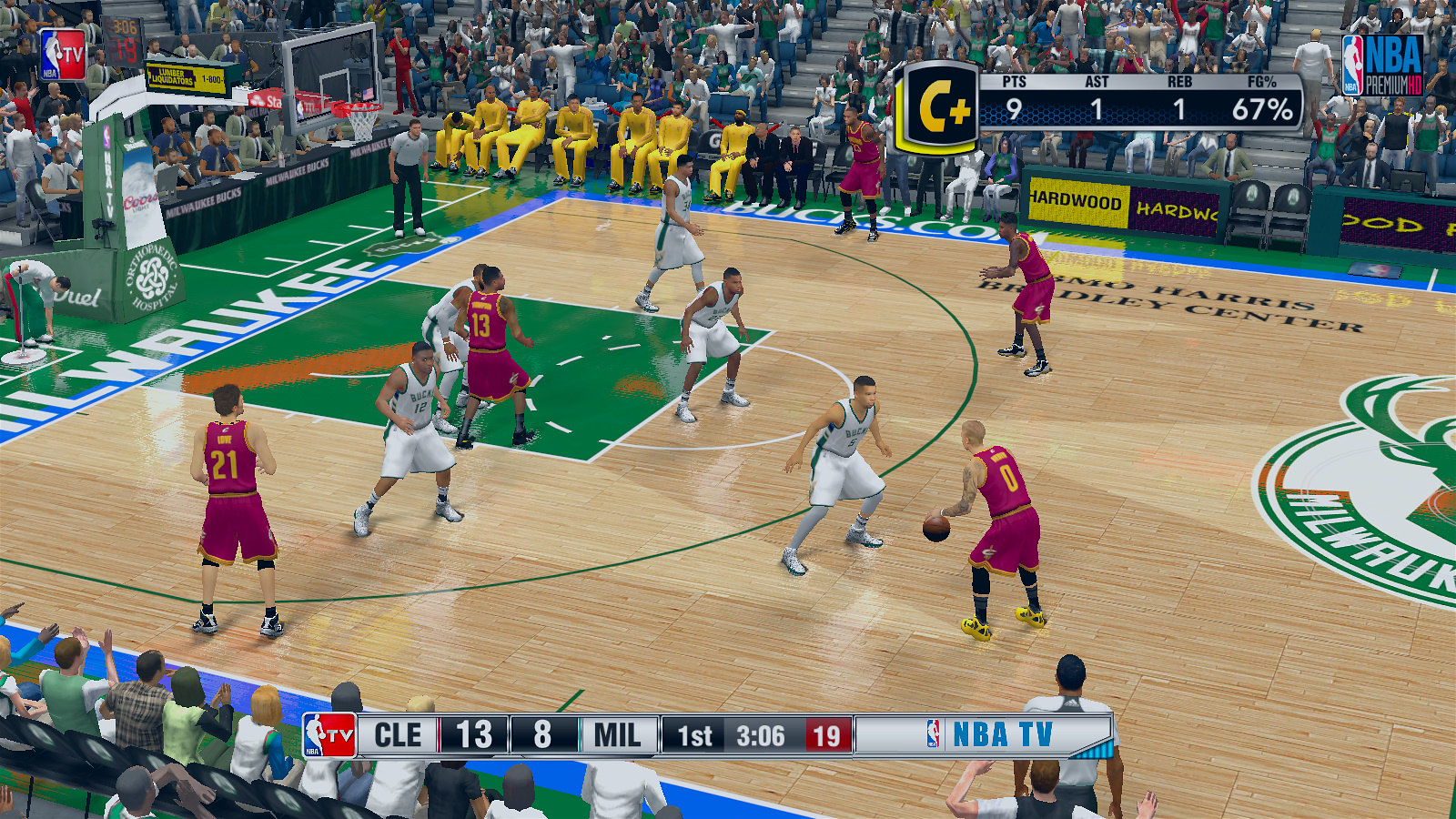This detailed caption is for an image taken from a PlayStation 2 era basketball video game, likely part of the NBA 2K series. The screenshot captures in-game action between the Milwaukee Bucks and the Cleveland Cavaliers. The Milwaukee team wears white jerseys with green stripes, while Cleveland sports purplish-pink jerseys with yellow lettering. It is the first quarter, with 3 minutes and 6 seconds left, and Cleveland leads 13-8. Notably, there's a scoreboard in the top right showing a player's stats: 9 points, 1 assist, 1 rebound, and a 67% field goal rate. The center court features the Milwaukee Bucks emblem, a deer, indicating the game is taking place in Milwaukee. The player from Cleveland is seen dribbling the ball at the top of the key, preparing to execute a play. The atmosphere is enhanced with visible crowds at the top and left of the screen, along with various advertising banners, including one from Hardwood. The bottom graphic overlays display the terms "CLE 13-8, MIL FIRST," highlighting NBA TV's broadcast. The vibrant scene encapsulates the nostalgic and competitive spirit of early 2000s basketball video games.